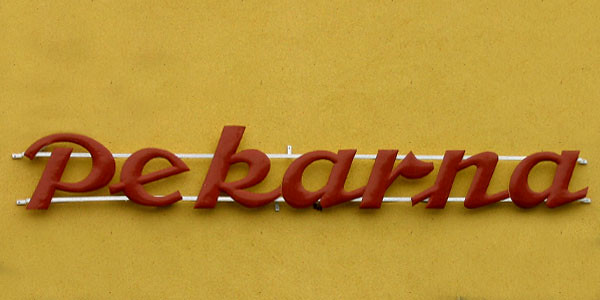Displayed prominently against a mustard-yellow wall, this signboard catches the eye with its bold presence. The sign, which reads 'Pekarna' in large red letters, is securely fastened to the building using two supportive bars. These bars are held in place by white brackets, each secured with screws on either end to ensure stability.

The text on the sign is an intriguing blend of script and print styles. Starting with a traditional, upright 'P', the lowercase 'e' features an extended horizontal line through the curve. The 'K' flows seamlessly in cursive, elegantly merging into the 'A', which is characterized by a sharp line at the bottom connecting it to the 'R'. The 'R' stands out in regular print but boasts a distinctive spike at the top. The 'N' is a standard printed form, leading into the final 'A', which intriguingly straddles the line between script and print styles.

Despite the unusual style of the lettering, the word 'Pekarna' is clearly displayed, though its meaning remains a mystery to the observer, suggesting that it might be a name or term uncommon in their locale.